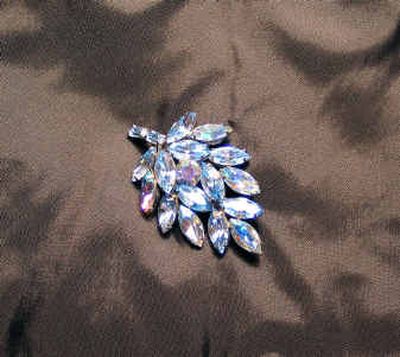The photograph showcases an intricate piece of jewelry, possibly a pendant or a single drop earring, artfully displayed on a rich brown velvet fabric that accentuates its elegance. The jewelry features an arrangement of approximately 20 marquise-cut gemstones, designed in a formation reminiscent of a pine cone or a cluster of leaves. These gemstones catch the light beautifully, with hues varying from blue to hints of pink and white. The overall composition is striking, with the high nap of the velvet fabric creating a dynamic light and dark gradient that enhances the jewelry’s luminous qualities.